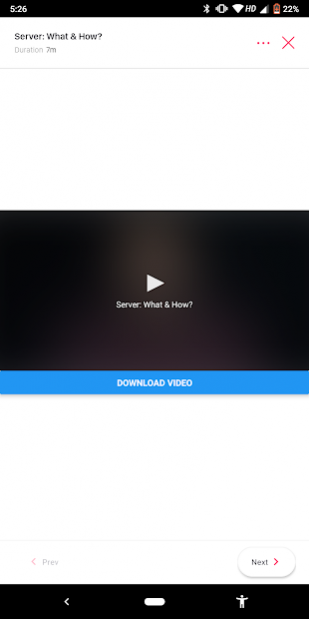The image is a screenshot taken on a smartphone. At the top left corner of the screen, the time is displayed as "5:26." Directly below the time, there is a bar labeled "Server: What and How" accompanied by a duration of seven minutes. On the right side of this top bar are two icons: a three-dotted menu button and an 'X' button for closing.

The background of the screenshot is primarily white, drawing attention to the centered paused video. The video features a large white play button, and below this, the text "Server: What and How" is prominently featured. At the bottom of the video frame, there is a blue bar containing white text that reads "Download Video."

Towards the lower section of the screenshot, there are two navigation buttons: the "Previous" button on the left and the "Next" button on the right. Finally, at the very bottom of the screenshot, a black navigation bar includes three icons: a back button on the left, a home button in the center, and a symbol on the right that resembles a person with their arm extended, possibly indicating accessibility or user options.